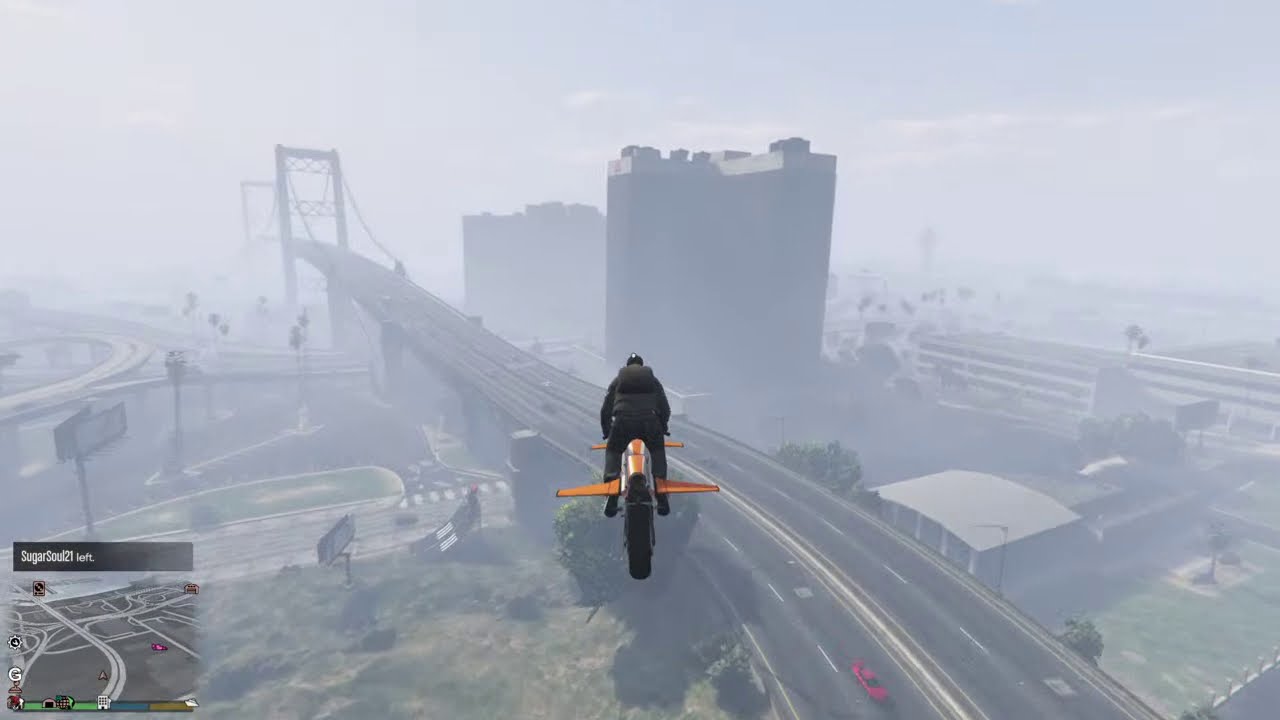In this detailed still image from the video game GTA 5 Online, the viewer is presented with a scene of a city shrouded in fog that obscures the details of the distant skyscrapers and highways. Central to the image is a character clad in a black outfit, wearing a black helmet and what appears to be a backpack, riding an orange and gray flying motorcycle with distinctive orange wings. The character faces away from the viewer as they soar high above the cityscape. Below the motorcycle, the city reveals a patchwork of grassy areas, streets, and a sprawling freeway system, with various buildings, billboards, and a suspension bridge stretching out into the mist. The scene is tinged with blue and gray hues, enhancing the foggy, atmospheric effect. In the lower left-hand corner of the image, the game interface displays the text "SugarSoul21 left," accompanied by a small map and a green, blue, and orange bar, indicating the player's position within the game environment.